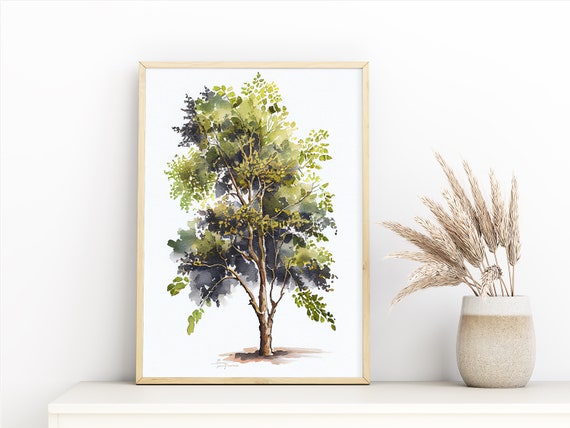This photograph depicts a tastefully arranged piece of home decor on a cream-colored desk set against a white wall. Centered on the desk is a delicate art print of a green-foliaged tree, framed by a thin, light cream wood frame. The white background of the print is accented with dark gray shadows behind the tree and brown shading at its base, adding depth to the depiction. To the right of the framed art print rests a stone or cement piece of pottery, characterized by its dark tan color and a lighter gray tan stripe near the top. This pot is filled with dried wheat stalks, some of which stand upright while others lean gracefully to the left, creating a charming rustic aesthetic.